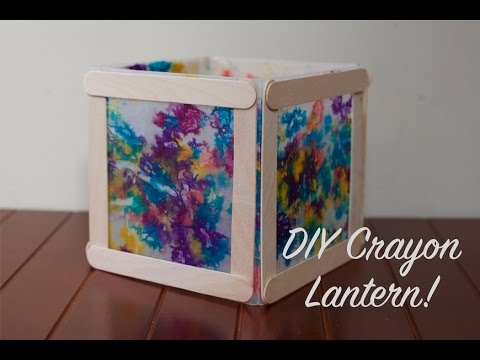This photograph showcases a DIY Crayon Lantern, captioned in cursive white text with an exclamation mark. Positioned on a reddish-brown wooden table with a white wall in the background, the image features a homemade lantern crafted from Popsicle sticks and melted crayon art. The top and bottom of the image are bordered with thin black strips. The lantern itself is a cube-like structure with an open top, constructed by gluing Popsicle sticks into squares and assembling them into a box. Each side of the box is filled with translucent wax paper, adorned with abstract, splotchy artwork in vibrant hues of purple, yellow, and blue, giving it a psychedelic, tie-dye appearance. This charming art project captures the creative essence of a child's craft, radiating a warm, handmade feel.